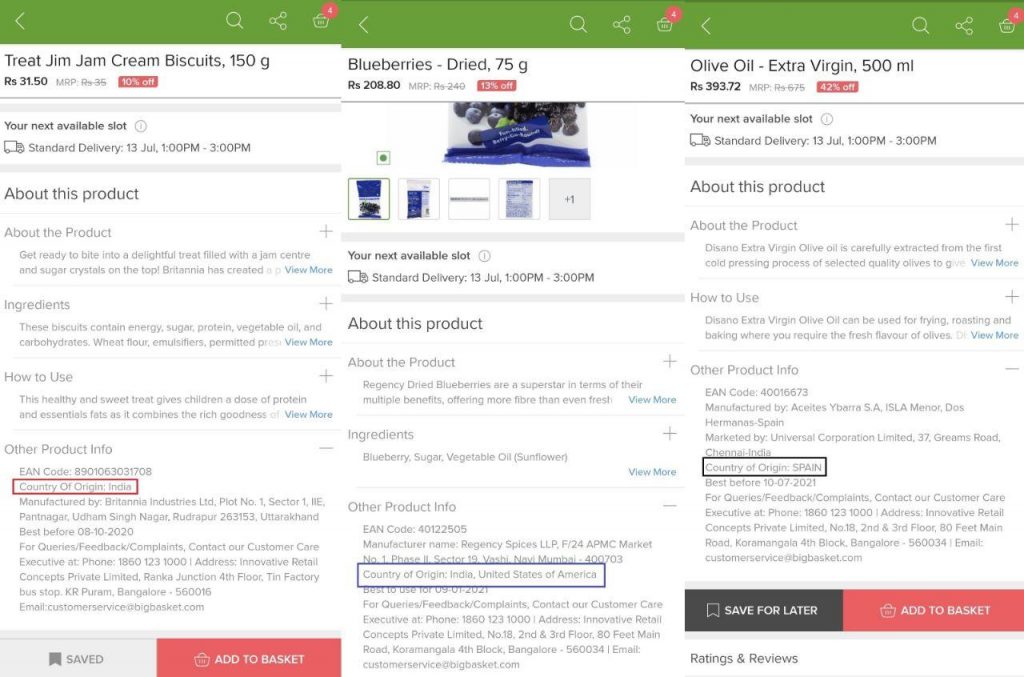This image showcases a set of three horizontally aligned screenshots from a grocery shopping app, each displaying a different product's details. At the top of all three screenshots, a green horizontal bar features a magnifying glass icon for search, a settings icon for app preferences, and a shopping basket icon with the number 4 inside a red circle, indicating the current items in the cart.

The first screenshot on the left highlights "Treat Jim Jam Cream Biscuits," packaged in a 150-gram quantity. 

The middle screenshot presents "Dried Blueberries" in a 75-gram pack. 

The rightmost screenshot displays "Extra Virgin Olive Oil" in a 500-milliliter bottle. 

All screens have a consistent white background with product-specific details in black or gray text, such as product descriptions, prices, delivery information, ingredients, and usage instructions—critical information for informed grocery shopping. 

Two of the screenshots feature functional buttons at the bottom: "Save for Later" to bookmark the product in light or dark gray, and "Add to Basket," a prominent red button with white text for immediate purchase.